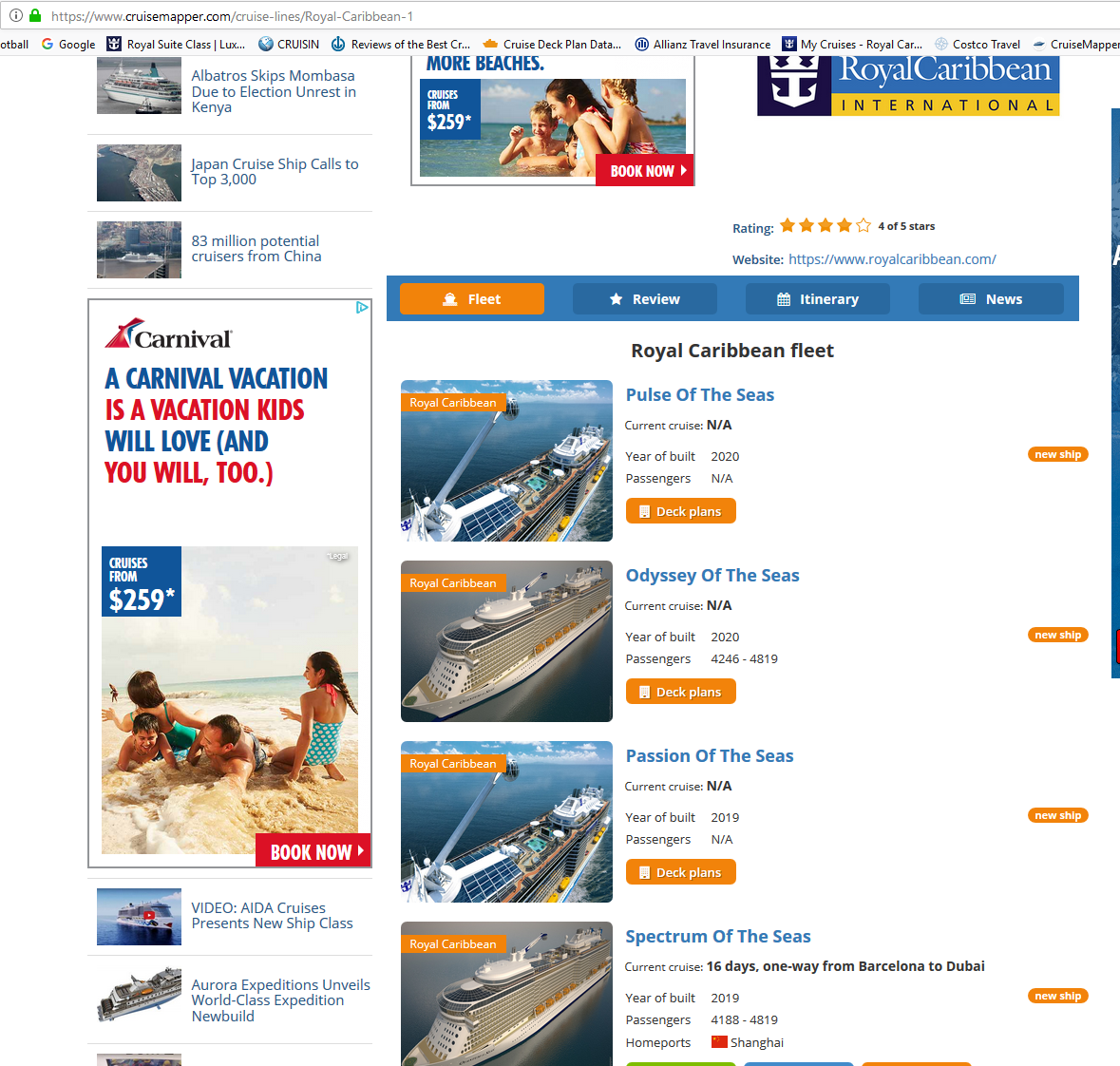The webpage displayed is a detailed cruise search platform called CruiseMapper.com, currently showcasing information about Royal Caribbean. Dominating the center of the page is a comprehensive list of Royal Caribbean’s fleet, featuring ships such as Pulse of the Seas, Odyssey of the Seas, Passion of the Seas, and Spectrum of the Seas. Each entry includes an image of the vessel, statistics detailing passenger capacity, the year of manufacture, and hyperlinks to detailed deck plans.

On the left side of the page, an advertisement for Carnival Cruises is visible, along with various links pertaining to other cruise lines and recent cruise-related news. At the top, the page provides an overview of Royal Caribbean, indicating a 4 out of 5 stars rating, and includes a link to the official Royal Caribbean website (royalcaribbean.com) alongside the Royal Caribbean logo.

Additionally, a prominent top-banner ad promotes cruise bookings with a starting price of $259, encouraging visitors to "book now." The browser’s bookmark bar is visible on the screen, displaying shortcuts to related resources such as Royal Suite Class for Royal Caribbean, general cruising reviews, cruise deck plan information, Alliance Travel Insurance, personal Royal Caribbean cruise reservations, Costco Travel, and Cruise Mapper.